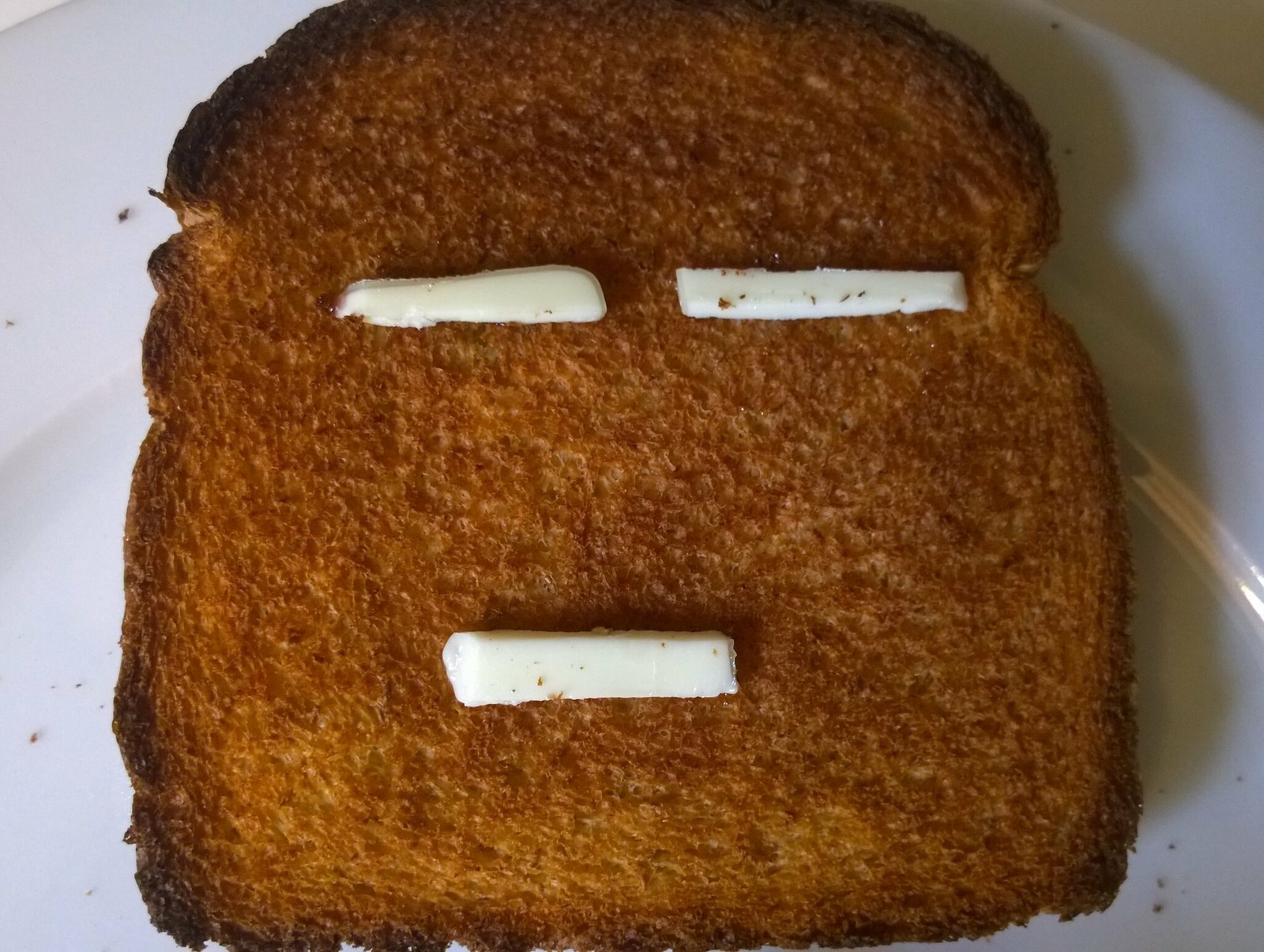The close-up image shows a single, well-toasted piece of bread on a flat white ceramic plate with a silver border. The toast is predominantly dark brown, with slightly burnt edges, indicating it was toasted for a prolonged period without being completely burnt. Surrounding the toast on the plate are several dark brown crumbs. On the top right-hand corner of the image, there's a small section revealing a dark mustardy surface underneath the plate. Arranged on the toast are three horizontal strips of white cheese, creatively placed to resemble a face with two slitty eyes and a slitty mouth, giving the toast a whimsical appearance.